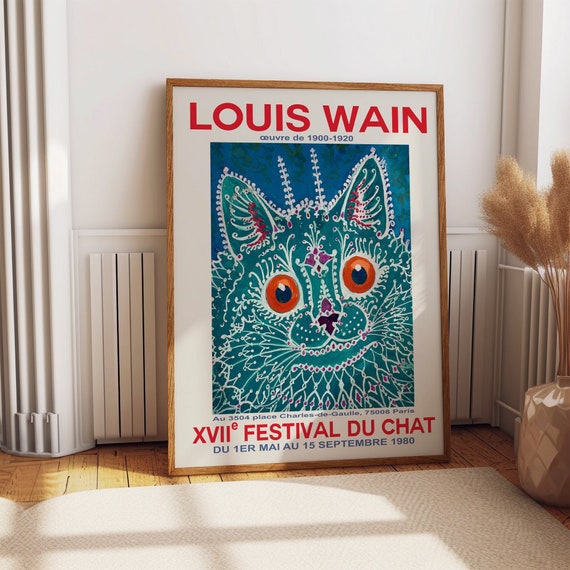The photograph, taken outdoors with natural lighting, is vertically rectangular and captures the interior of someone's home. The focus is a framed poster leaning against a white wall, with the upper right section revealing light streaming from off-camera, potentially from a nearby window. Adjacent to the poster on the right side is a brown planter holding wheat-colored plants with fuzzy tips. The setting includes a wooden floor adorned with a white rug that reflects the light and shadows from the window.

The poster is encased in a brown wooden frame and stands against the wall at a slight slant. The poster itself features a predominantly white background with a striking blue vertical rectangle in the center. At the top, in bold red letters, it reads "Louis Wain." Beneath this, blue text includes the dates "1900 to 1920." The bottom part of the poster showcases "XVII Festival du Chat" in red Roman numerals, followed by details in smaller blue lettering that mark the event from "Du 1er Mai au 15 September 1980."

The centerpiece artwork on the poster is a detailed cat face rendered in teal blue with intricate white lace-like patterns throughout. The eyes of the cat are vibrant orange with blue centers, and its nose has a purple tint. Additional text at the bottom includes an address in Paris, further emphasizing the poster's cultural and historical context.